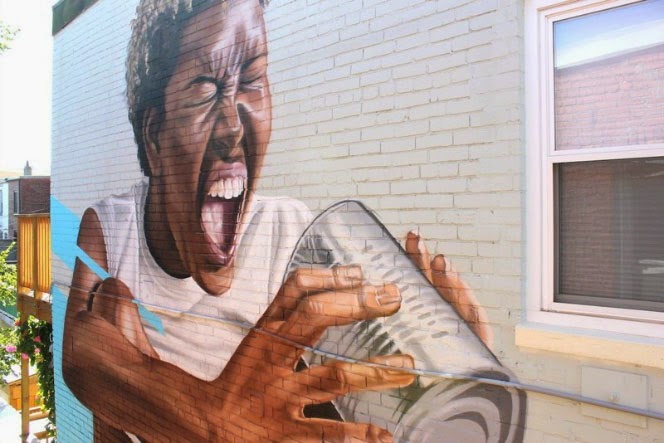This captivating rectangular photograph features a detailed mural painted on the off-white brick side of a building. The central focus of the mural is a dark-skinned child, possibly a girl, captured in an emotionally intense moment. Dressed in a sleeveless white t-shirt, the child is depicted sitting with knees up, clutching a tin can, into which they appear to be screaming with eyes tightly shut. The child's expressive face, with an open mouth and visible upper teeth, is partially cropped at the top of the image, cutting off just above the forehead.

To the right of the mural, a bright white window frame adds contrast to the wall. The left side of the image features a glimpse of a balcony adorned with some flowering plants, hinting at greenery. An electrical line runs across the scene, adding to the urban texture. The photograph captures the side of the building in its entirety, suggesting this painting is a prominent feature, likely situated a few floors above street level, reminiscent of a sophisticated piece of street art and graffiti combined. The backdrop includes a white sky, enhancing the mural’s vividness and the building’s architectural details.